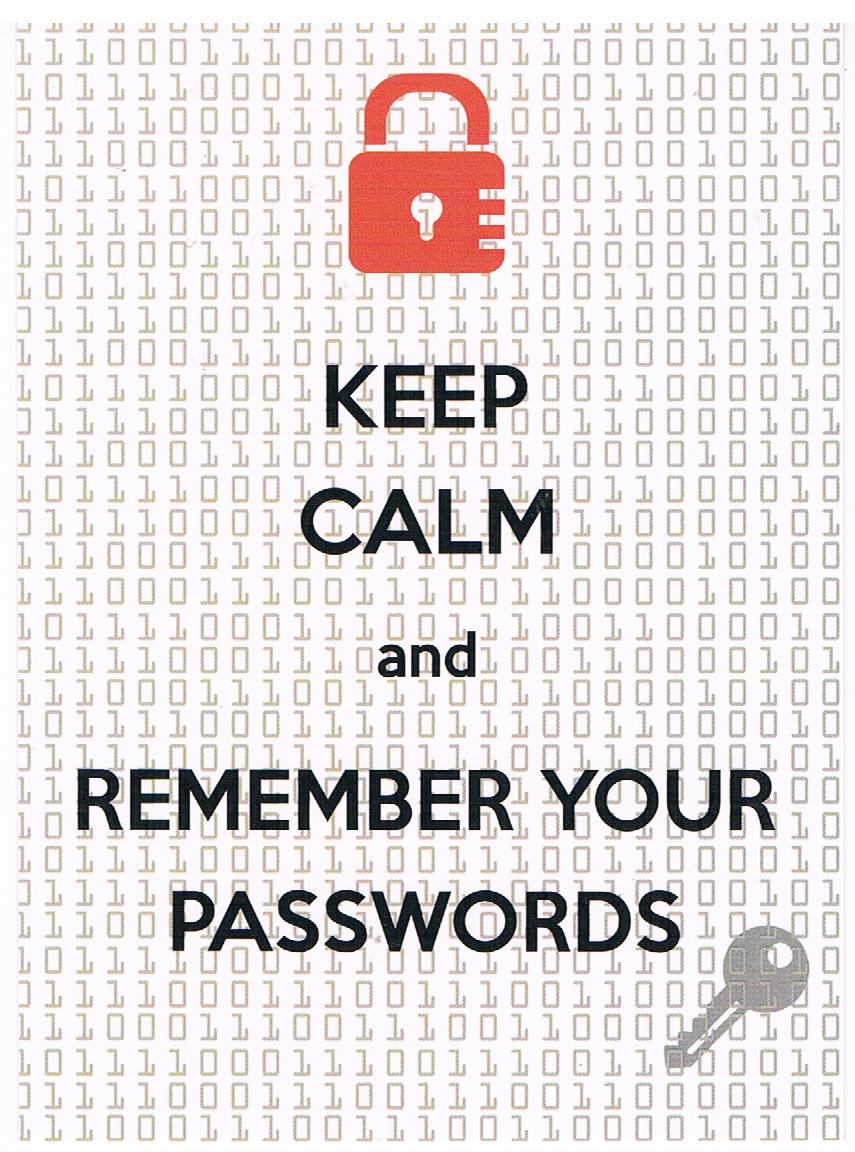The poster features a light backdrop adorned with a detailed pattern of ones and zeros in shades of light brownish-gray and white. At the top center, there's a cartoon-style red lock with a keyhole that allows a glimpse of the binary code behind it. Boldly centered below the lock, the phrase "KEEP CALM" is displayed in large, all-capital letters. The word "AND" follows, in slightly smaller but still prominent lowercase text, before concluding with the words "REMEMBER YOUR PASSWORDS," also in uppercase. In the lower right corner, a silver key is depicted, oriented downward and designed to fit the lock above. The overall design melds together cybersecurity themes with a reassuring message about password safety.